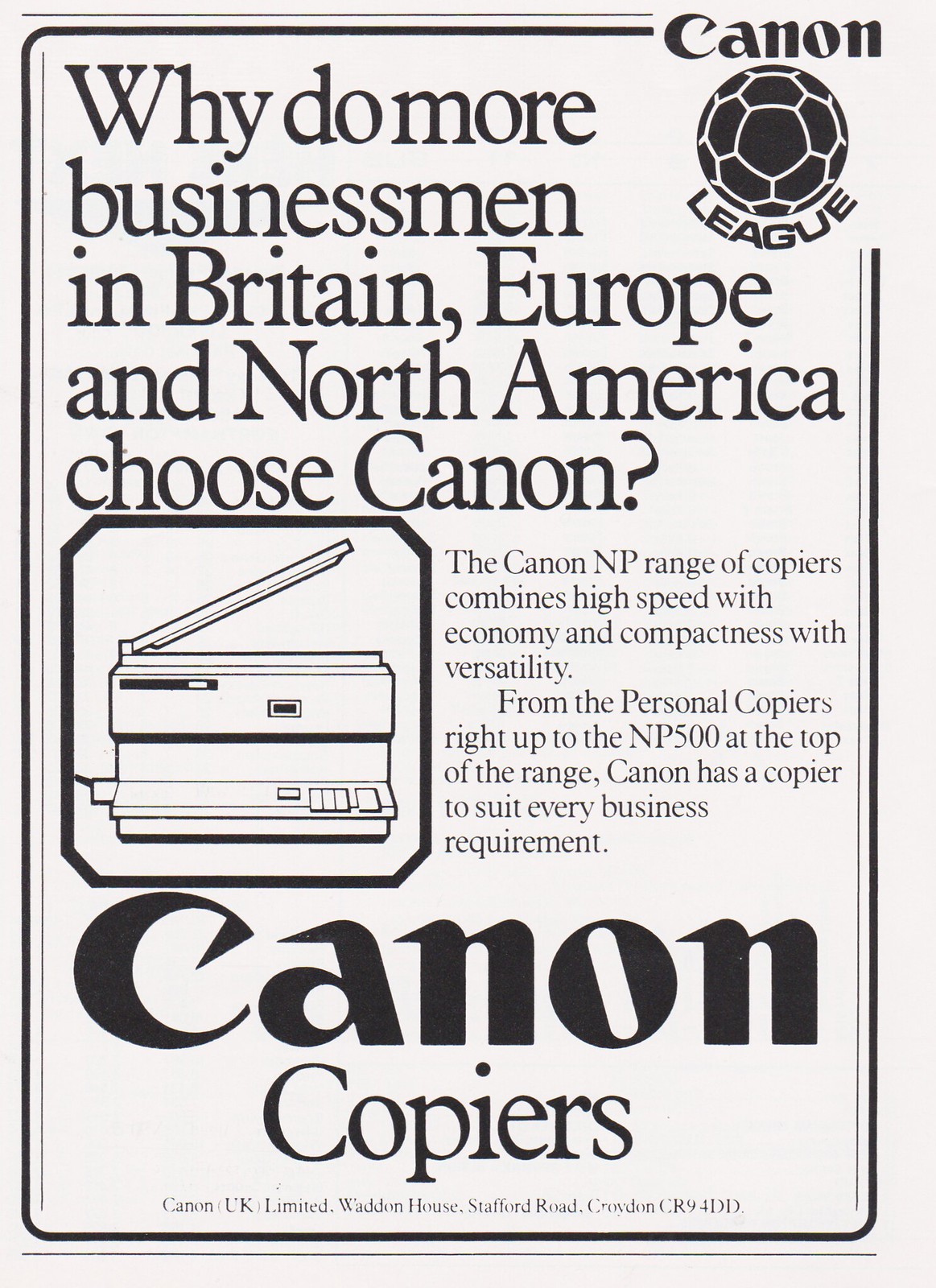This black and white newspaper advertisement for Canon copiers prominently features a Canon League soccer ball design in the upper right-hand corner. To the left of this logo, the headline reads, "Why do more businessmen in Britain, Europe, and North America choose Canon?" Below the headline is an image of a Canon photocopy machine with its top likely open. Adjacent to the image, the ad highlights the Canon NP range of copiers, emphasizing their high speed, economy, compactness, and versatility. It states, "From the personal copiers right up to the NP 500 at the top of the range, Canon has a copier to suit every business requirement." The lower section of the ad displays the phrase "Canon copiers" in bold, followed by the contact information: "Canon UK Limited, Wadden House, Stafford Road, Croydon, CR 9 4DD." The Canon logo is prominently featured at the bottom of the advertisement.